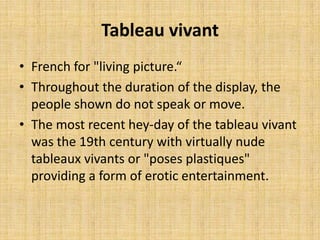The image is a horizontal slide presentation with a textured tan background resembling wicker or linen. At the top, centered and in bold, is the title "Tableau Vivant." Below the title are three black text bullet points, left-aligned. The first bullet point reads, "French for 'living picture.'" The second bullet point states, "Throughout the duration of the display, the people do not speak or move." The third bullet point explains, "The most recent heyday of the Tableau Vivant was the 19th century, with virtually nude Tableau Vivants or 'Pose Plastique' providing a form of erotic entertainment."